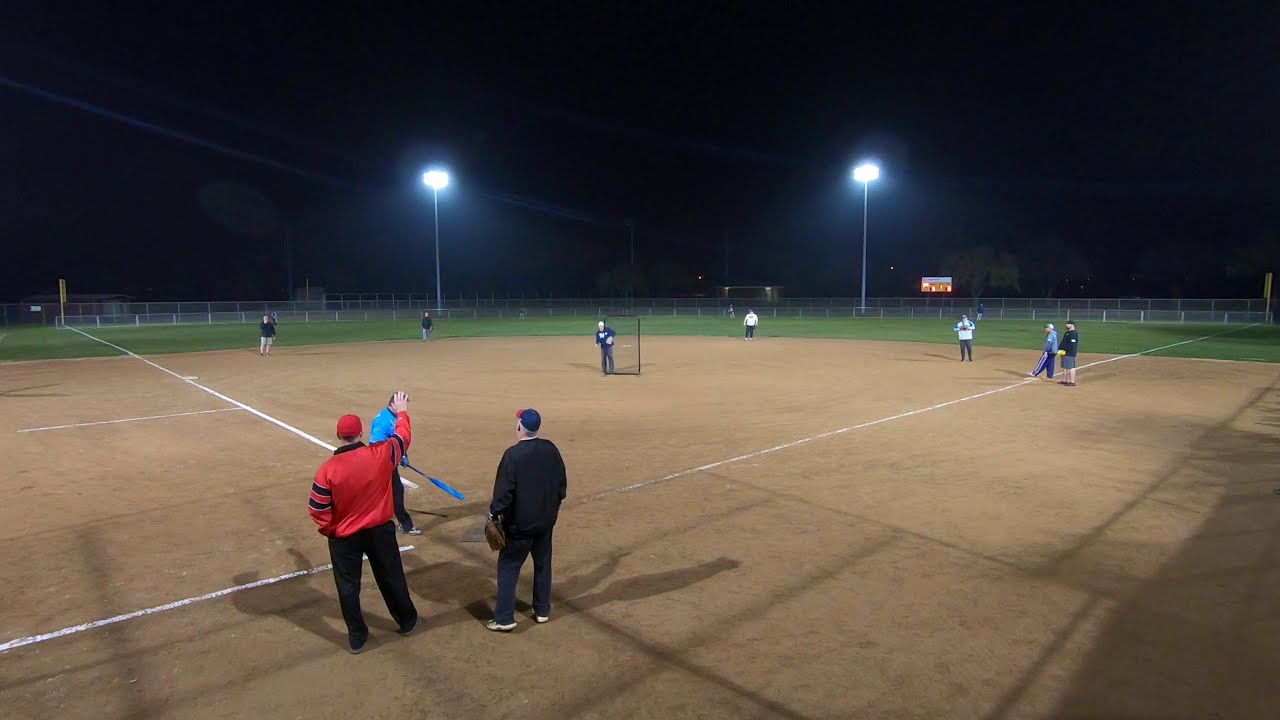In this nighttime photograph of a baseball diamond, the scene is illuminated by two tall streetlights against a dark sky. The infield is made of dirt with white painted baselines, while the outfield boasts green grass enclosed by a curved fence. Near home plate, an umpire wearing black slacks, a red jacket, and a red ball cap, raises his right arm. Standing next to him is the catcher, dressed in black pants and a black shirt, and holding a glove in his left hand. The batter, sporting a blue jacket and holding a matching blue bat, is poised to hit.

Beyond home plate, the field hosts ten additional players in varied positions. Visible are players covering third base, shortstop, pitcher (shielded by a net behind him), second base, and first base. A coach or another player stands on first base, likely assisting a runner. Across the image, the players’ uniforms feature a mix of blue, white, and semi-blue tops. The color palette of the scene includes shades of brown, green, black, red, blue, beige, tan, gray, white, and yellow. There are no visible spectators, and the overall framing of the photograph is a horizontal rectangle with the outfield spanning the center of the horizon, and the two streetlights positioned towards the top center of the image.